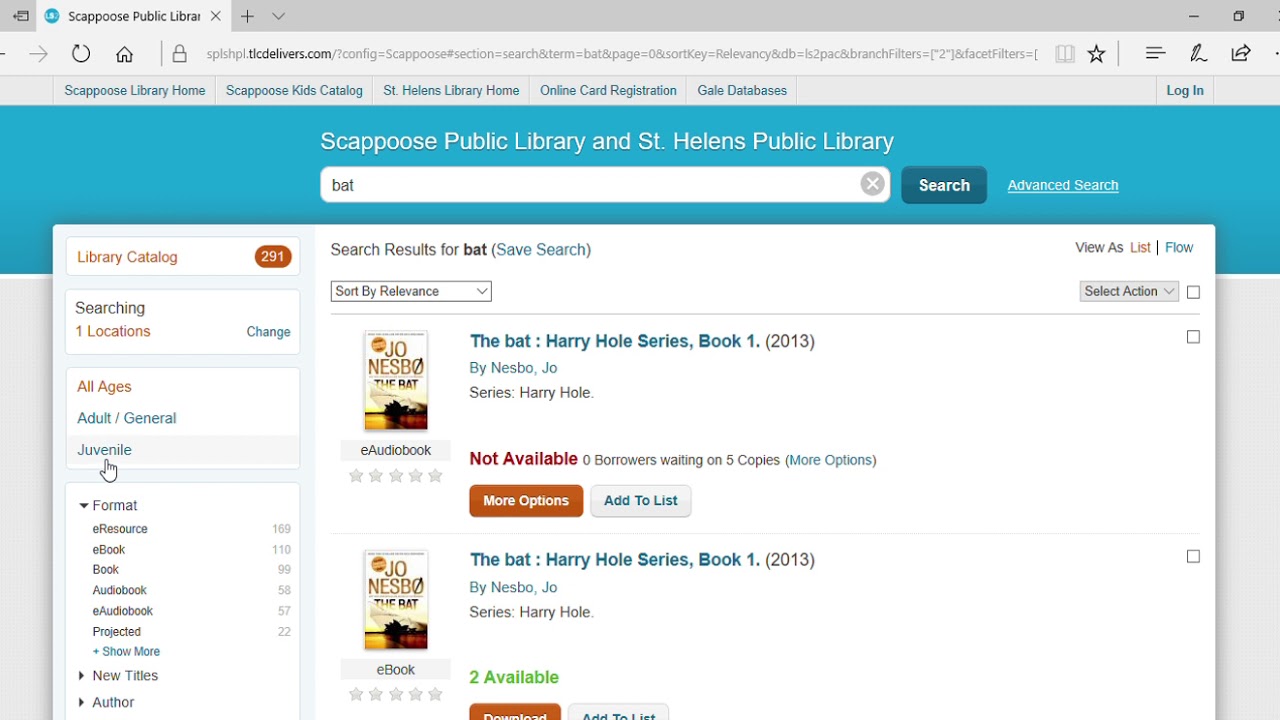On the screen, a tab in the browser displays "Scappoose Public Library" indicating their website is open. The navigation menu features several options: "Scappoose Library," "Scappoose Kids Catalog," "St. Helens Library," "Home," "Online Card Registration," "Gale Database," and "Login." Below the menu, the header reiterates "Scappoose Public Library and St. Helens Public Library." 

Centered on the page is a search bar with the term "BAT" typed inside. To the right of the search bar are buttons for "Search" and "Advanced Search." Next to these, underlined text reads "BAT." The left side of the page shows the library catalog status, indicating "291" and specifying it is "Searching one location." Options to "Change" the location or filter by age category ("All Ages," "Adult," "Juvenile") are available. 

A cursor, appearing as a hand, is pointed at the "Juvenile" filter. Below this, the search results for "BAT" are displayed: "The BAT, Harry Hole Series, Book 1" by Nesbo (not "Nespo"), Joe. The series title "Harry Hole" is noted, but the book’s status is marked as "not available."

Each element of the library website and search interface is meticulously described, creating a clear picture of the online experience.